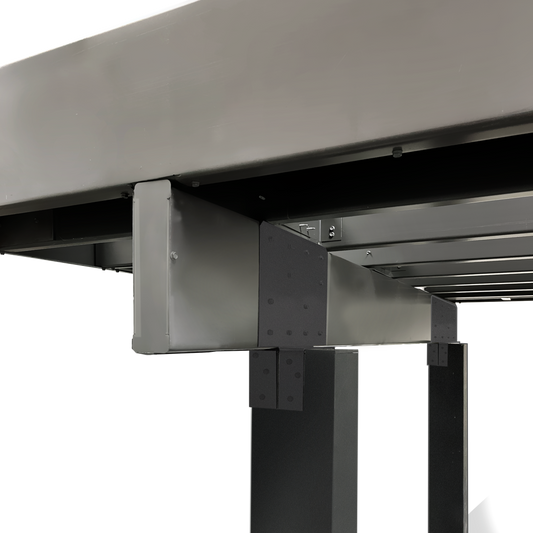The close-up image showcases a section of a sturdy, metal picnic table against an artificially white background, likely edited to remove real surroundings. The table features a large, metallic surface composed of grey slats, which are supported by multiple grey and silvery beams running horizontally. Below these beams, a single support beam extends perpendicularly, intersecting the horizontal ones. Supporting this structure are two black metal legs, giving it a robust appearance. The table seems designed for practicality, potentially allowing the legs to fold for easy storage and mobility. Several black bolts secure the beams, emphasizing the table's strong and durable construction. Overall, the image highlights a functional and heavily built metal picnic table, although only a small portion of it is visible.